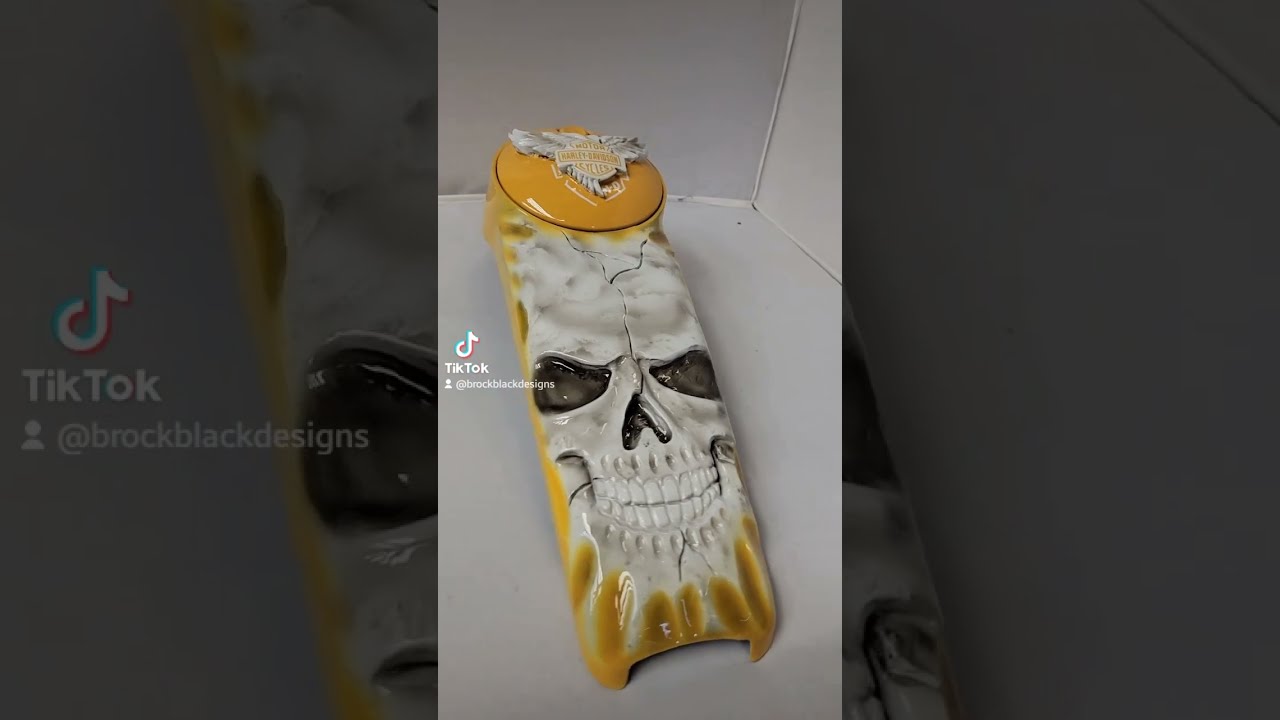This image appears to be a snapshot from a TikTok video by Brock Black Designs, featuring a detailed ceramic decorative piece. The main body is a rectangular pottery item vividly depicting a human skull in white with lifelike cracks running through it, suggesting it might have been broken and meticulously repaired. The skull's eyes are black, giving it an intense stare, and its teeth are prominently displayed at the bottom. The piece is framed with bright orange edges that hint at a hellfire, brimstone aesthetic, adding a dramatic flair. On top rests a round lid adorned with the iconic Harley-Davidson logo, indicative of a biker theme, with the logo crafted in gray and orange hues. The background of the image is minimalistic, with a white floor and two white walls, accentuating the boldness of the piece. Additionally, the left side of the image shows the TikTok logo and, beneath it, white text identifying the content producer. On either side of the primary image are zoomed-in gray elements, adding depth to the presentation of this high-quality, meticulously crafted ceramic item, which could serve as a striking display piece in any living space.